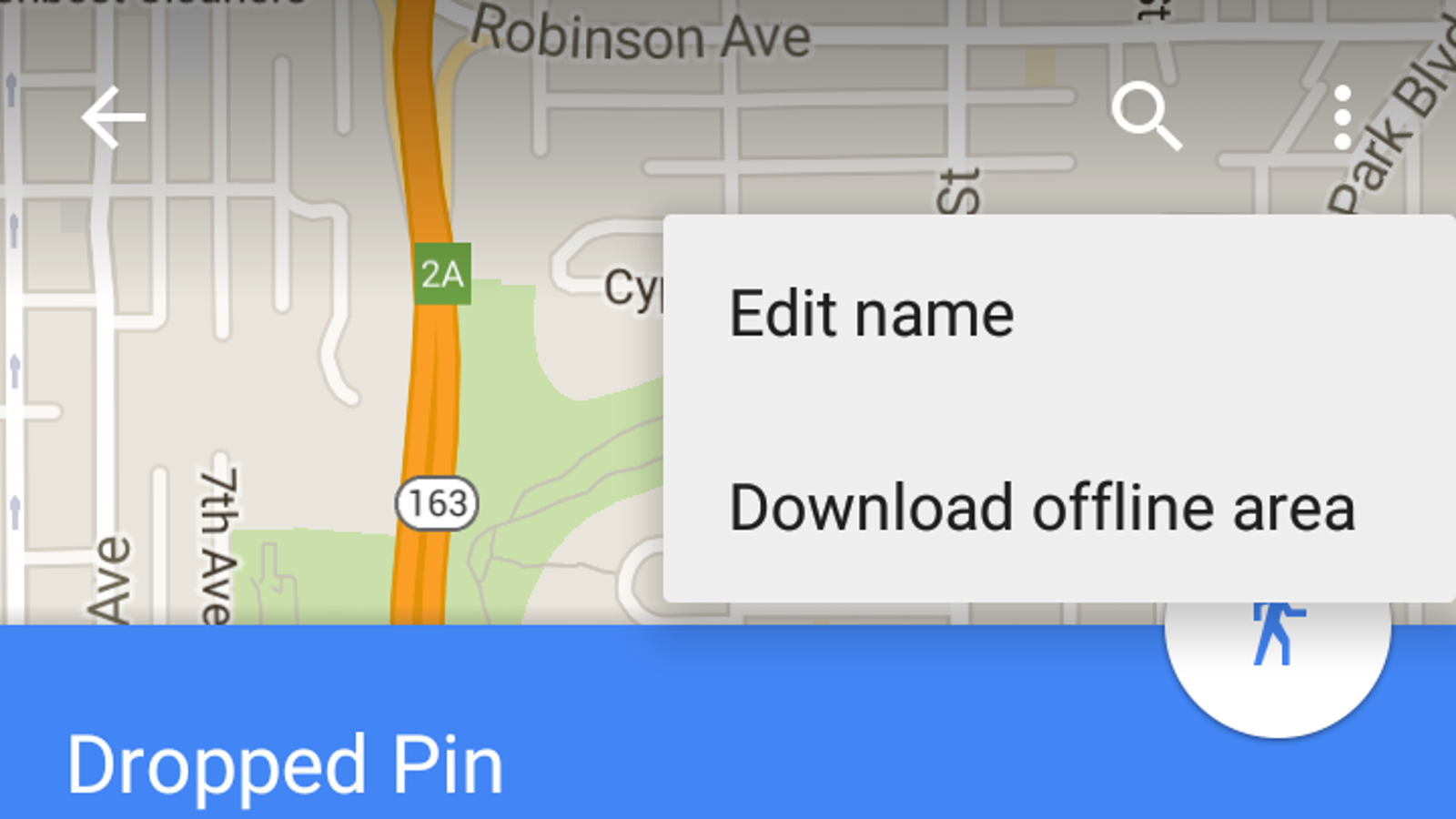This image is a detailed screenshot from Google Maps, showcasing a focused view of a specific area. The screenshot is landscape-oriented and nearly twice as wide as it is high. 

Predominantly, the top 75% of the image features a busy road map on a light gray background, with the roads marked in white. In the upper left corner, there's a white arrow pointing left, and in the upper right but not fully in the corner, there are two familiar icons: a magnifying glass (search icon) and three vertically stacked small white circles.

A significant landmark is an expressway that runs vertically from near the bottom to the top of the image. This highway is represented by an orange-yellow double-thick line which bends slightly. Near the bottom of the expressway, a white oval contains the number "163," indicating the route number. Further up, a green circle with the inscription "2A" marks another route.

Several road names are visible on the map: "Robinson Ave" is stated near the top center, while "7th Ave" appears tilted 90 degrees on the left side. 

Towards the lower right portion of the map, a white rectangular box obscures part of the image. This box contains two lines of text: "Edit name" in black and "Download offline area" beneath it. This box covers a considerable part of the map.

On the lower part of the image, flanking both sides of the expressway, are light green areas that resemble parks. The entire bottom quarter of the image is overlaid with a medium blue background. In the lower-left corner of this blue section is the text "Dropped pin" in a fairly large font. 

Towards the middle-right of this blue section, there is a white circle that is partially embedded into the blue background. This circle, which sits on top of the map, contains a blue icon of a person walking. However, part of this walking figure's head is obscured by the aforementioned white rectangular box that says "Download offline area."

This layered composition reveals an intricate blend of map details and interface elements characteristic of Google Maps, highlighting various navigational and functional features.